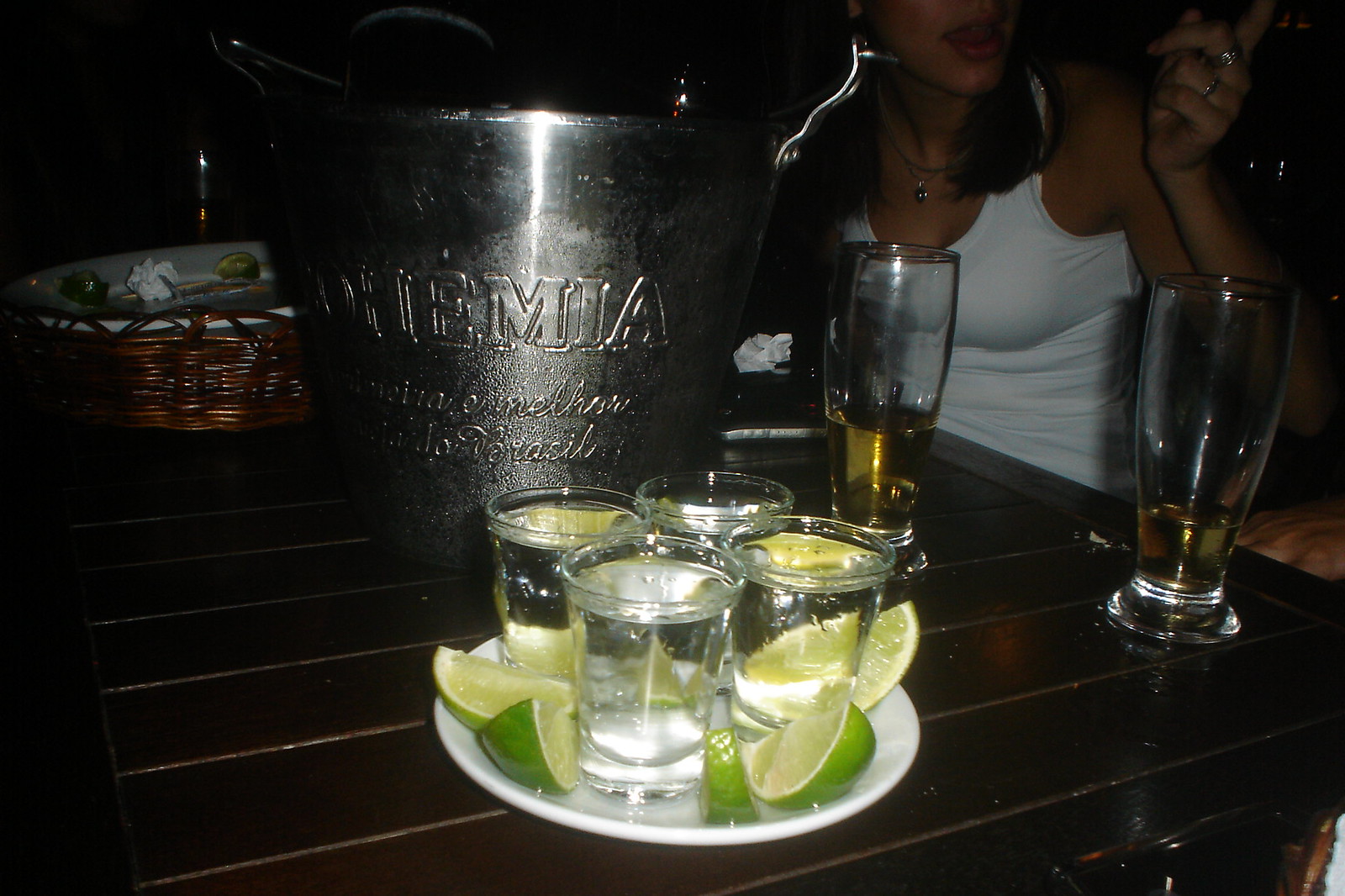In the dimly-lit atmosphere of a bar or restaurant, a close-up image captures a lively scene centered around a black-stained wooden table. Dominating the right side of the frame is a woman with olive skin, pink lipstick, and short brown hair, though the photograph cuts off the top of her head. She is animatedly talking with her mouth agape and tongue out. She dons a white, short-sleeved dress accentuated with two silver rings and a pendant necklace.

The table is set for a spirited night out, featuring a small ceramic white plate surrounded by clear shot glasses filled with a clear liquid, likely vodka or tequila, accompanied by lime wedges placed around the rim. Nearby, four clear glasses with yellow liquid, possibly beer or wine, are nearly emptied. Highlighting the tabletop decor is a silver and dark gray ice bucket with intricate engraving and embroidery, possibly holding bottles of alcohol just peeking out. Adjacent to the bucket, a dark brown wicker basket holds miscellaneous items, possibly leftovers or snacks like pretzels or breadsticks.

The ambiance suggests a setting where the woman, along with unseen companions, is poised to enjoy shots, evident from the array of clear and colorful beverages, surrounded by the casual disarray of a convivial time.